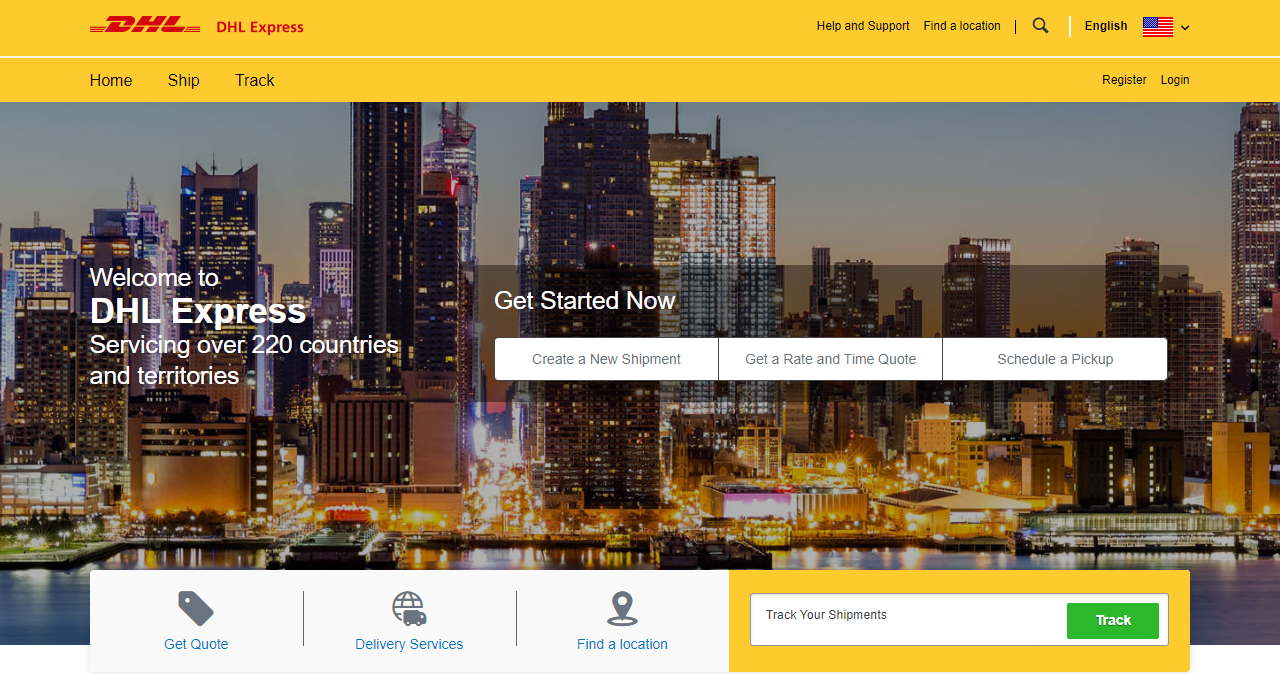This image is a screen capture from a computer or laptop monitor, showcasing the homepage of the DHL Express website. The website interface is rectangular, with the longer side oriented horizontally. 

At the top, there are two rectangular banners in varying shades of orangey-yellow. On the upper right of the banners, the text “Help and Support” appears in blue letters. Next to it, there is an icon of a magnifying glass accompanied by the phrase “Find a Location.” Further right, there is a selection drop-down that says “English,” next to an icon of the US flag.

Below these banners, there is another horizontal, solid fill border with black text. It features navigation options: “Home,” “Ship,” “Track,” and towards the right side, options to “Register” and “Login.” 

Prominently displayed below the navigation menu is a color photograph capturing a cityscape at dusk. The image depicts numerous skyscrapers with their windows warmly lit. Superimposed on this image, in large white text, is the message: "Welcome to DHL Express, servicing over 220 countries and territories." Just below this statement, there are clickable options to “Get Started Now,” including actions to “Create a New Shipment,” “Get a Rate and Time Quote,” or “Schedule a Pickup.”

At the bottom of the screen capture, additional options are listed in smaller text: “Get a Quote,” “Delivery Services,” “Find a Location,” and “Track Your Shipment.”